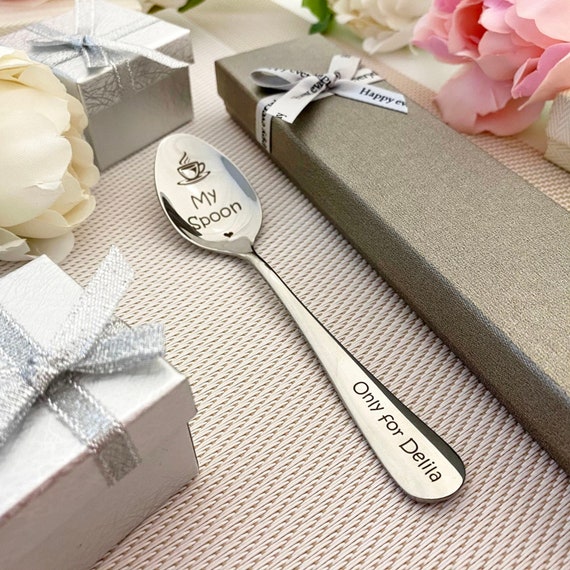The image portrays a beautifully set table for a birthday celebration, possibly for an adult named Delilah. Dominating the foreground is a silver spoon labeled "My Spoon," featuring a coffee cup illustration in the bowl and the inscription "Only for Delilah" on the handle. The table brims with festivity, adorned with wrapped presents, vibrant flowers, and a long grey box tied with a ribbon, which partially displays the message "Happy Birthday." A delicate pink flower graces the top right corner, adding to the celebratory atmosphere, suggesting that a joyous occasion is about to unfold.